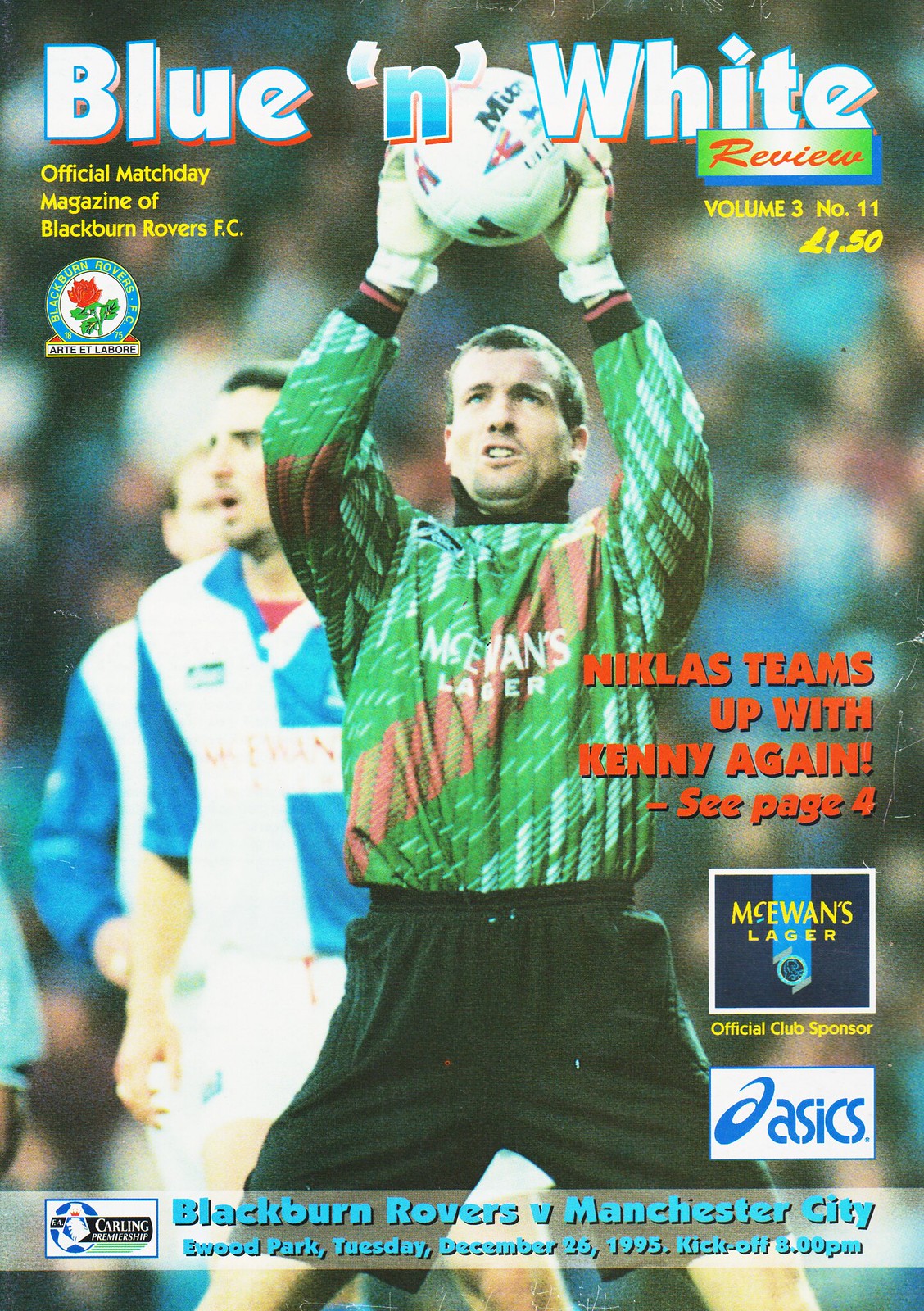The cover of the official match day magazine of Blackburn Rovers FC prominently features the title "Blue and White Review" in striking white font with a blue background. The subtitle, "official match day magazine of Blackburn Rovers FC," is placed just below and is accompanied by the team's iconic logo, a blue-bordered circle with a red rose at its center. The main image captures a moment of anticipation, showcasing a goalkeeper dressed in a long-sleeved green shirt and black shorts. His gloved hands hold a soccer ball aloft as he looks towards the sky, signaling the start of the game. Behind him, two players in blue and white uniforms are visible. The right side of the cover includes the text, "Nicholas teams up with Kenny again – see page four," in bold red print. Below this, an ad for McEwen's Lager, the official club sponsor, is noticeable. The bottom panel details the match information: "Blackburn Rovers vs. Manchester City, Brood Park, Tuesday, December 6, 1995, kickoff at 5:30 p.m." Additionally, the tagline "Volume 3, Number 11" and "L 150" are featured, along with the ASICS logo, marking its association with the event.